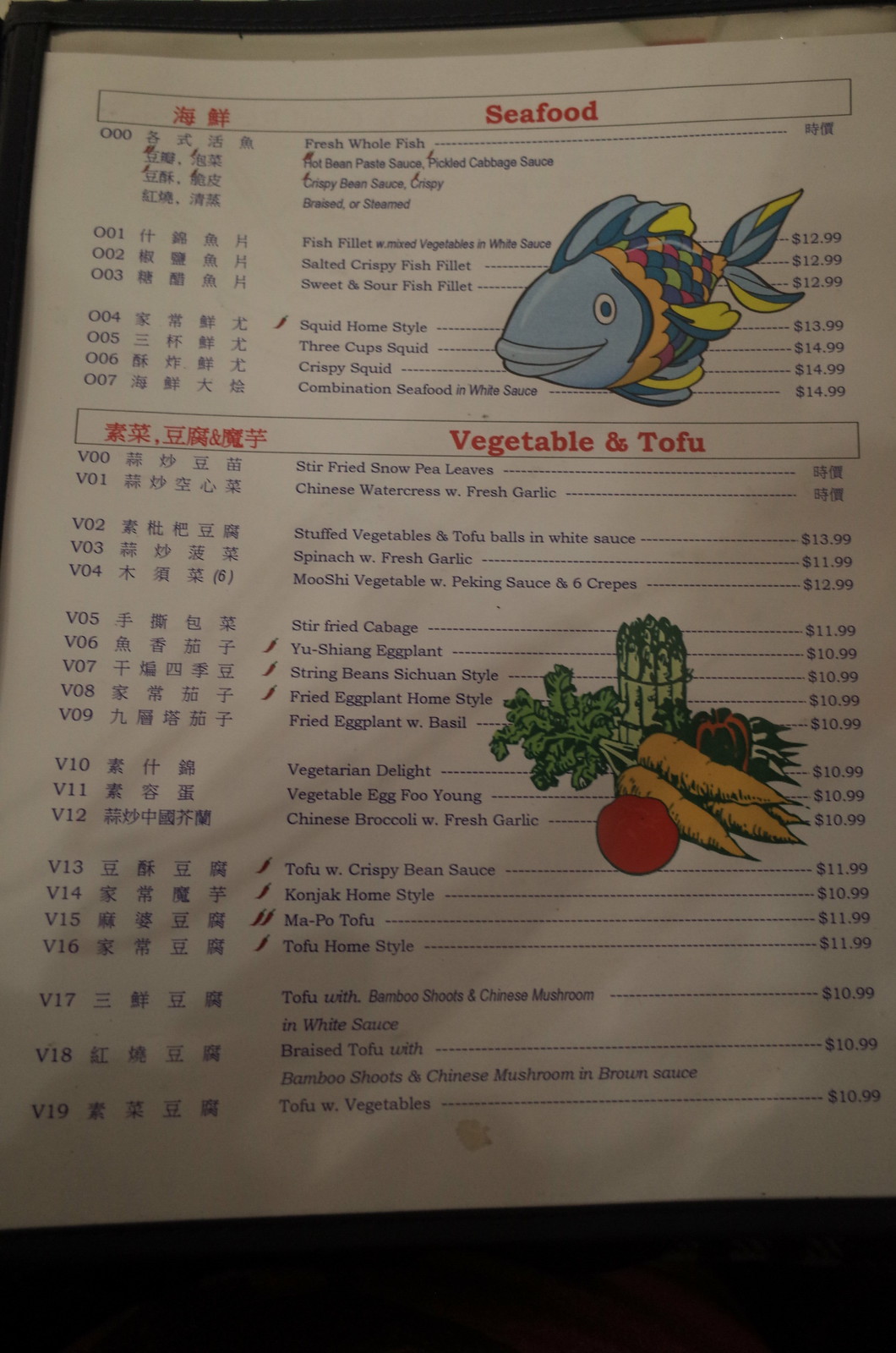At the top of the paper menu, there is a long, thin rectangle with the word "Seafood" prominently displayed in red letters. Below this, a vibrant, detailed illustration of a fish faces left. The fish is depicted with big blue lips, a white eye with a black pupil, and a body adorned with a kaleidoscope of scales in shades of yellow, green, blue, orange, and red. The tail is a blend of yellow, gray, and blue. 

To the right of the fish illustration, a list of prices is presented, ranging from $12.99 to $14.99. On the left side of this section, the names of seafood dishes like "Fish Fillet" and "Salted Crispy Fish Fillet" are listed, accompanied by characters in a foreign language.

Beneath the fish section, another rectangle features the heading "Vegetable and Tofu" in red letters. Below this heading, a charming illustration depicts a variety of vegetables. Orange carrots with green tops point downward to the right, while a bundle of asparagus stands upright in the background. A tomato is positioned in the bottom left corner of the illustration. 

Adjacent to this artwork, the names of vegetable dishes, such as "Stir Fry" and "Snow Pea Leaves," are listed on the left. The right side displays their corresponding prices, ranging from $13.99 at the top to $10.99 at the bottom. Additional characters in a foreign language are also present on the far left side of this section.